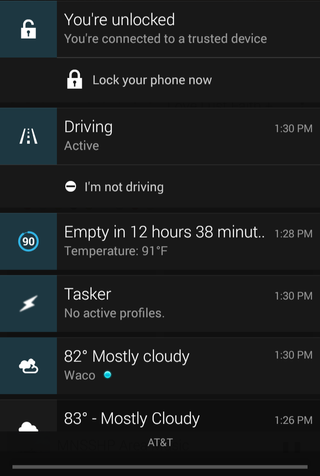The image shows a smartphone screen featuring various options and statuses, each separated by fine grey lines. The first icon, set against a blue background, depicts an unlocked lock. To the right, the text reads, "You're unlocked, connected to a trusted device," with an option below to "lock your phone now." The next icon is a road symbol on a blue background, accompanied by the word "Driving" with "active" status. Directly underneath is an option labeled "I'm not driving." The third icon is a blue circle with the number "90" inside, displaying text that reads, "Empty in 12 hours, 38 minutes, temperature 91˚F." Following this is a lightning bolt icon on a blue background, with the text "Tasker, no active profiles" beside it. Next is a cloud icon indicating the weather, which reads "82˚, mostly cloudy, Waco." Another cloud icon, this time against a grey background, shows "83˚, mostly cloudy." At the very bottom center of the image, it shows "AT&T" as the network provider.